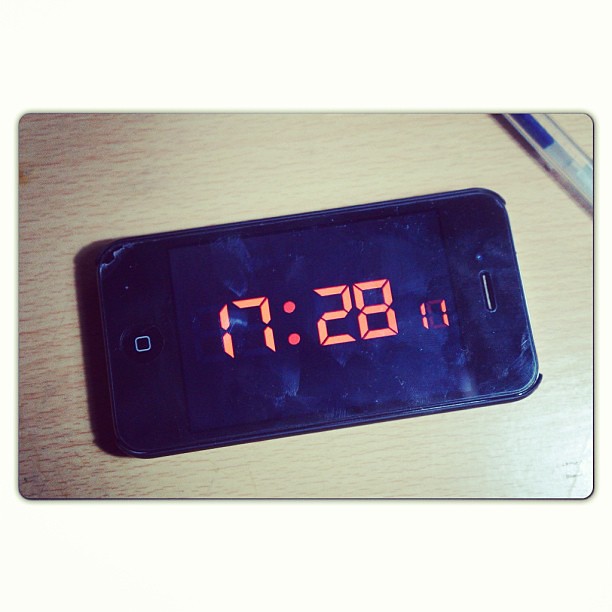The image features a black, older model iPhone with a home button displaying the time "17:28:11" in orange digital numerals. The phone is situated on a light-colored wooden desk or countertop with a distinct texture, suggesting it may be real wood or a high-quality imitation. The iPhone's screen protector is visibly cracked in the upper left corner, and there are minor scuff marks on the upper right corner of the phone. Partially visible in the upper right corner of the image is a ballpoint pen with blue ink, positioned at approximately a 45-degree angle. The pen extends past the edges of the image, with neither end visible. The overall photograph appears to have a dark Instagram-like filter, adding a subtle shadow effect to the scene. This image is printed on a rectangular, rounded-corner mouse pad.